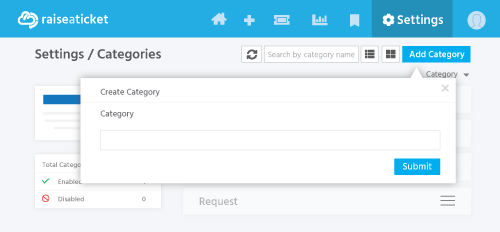The image depicts a website interface focused on a ticketing system. The main section features a distinctly white and blue theme, with an icon resembling a cloud with a hint of blue. The current section displayed is 'Settings' under 'Settings/Categories'. The user is prompted to search by category name and given the option to add a new category.

When the 'Add a Category' button is clicked, a pop-up appears, labeled 'Create a Category', where users can input the name of a new category and submit it. Upon submission, the user is returned to the original settings page, which is partially obscured by the pop-up.

In the bottom left of the interface, there is an area labeled 'Total', the rest of which is hidden, with an 'Enabled' option that has a green check mark indicating it is active. Below the pop-up box, there is a section titled 'Requests' featuring three horizontal lines, suggesting a clickable menu that likely contains various categories.

Adjacent to the 'Raise a Ticket' icon at the top, there are other icons that provide additional support features. On the far right side of the interface, there appears to be a link or icon for customer service connection.